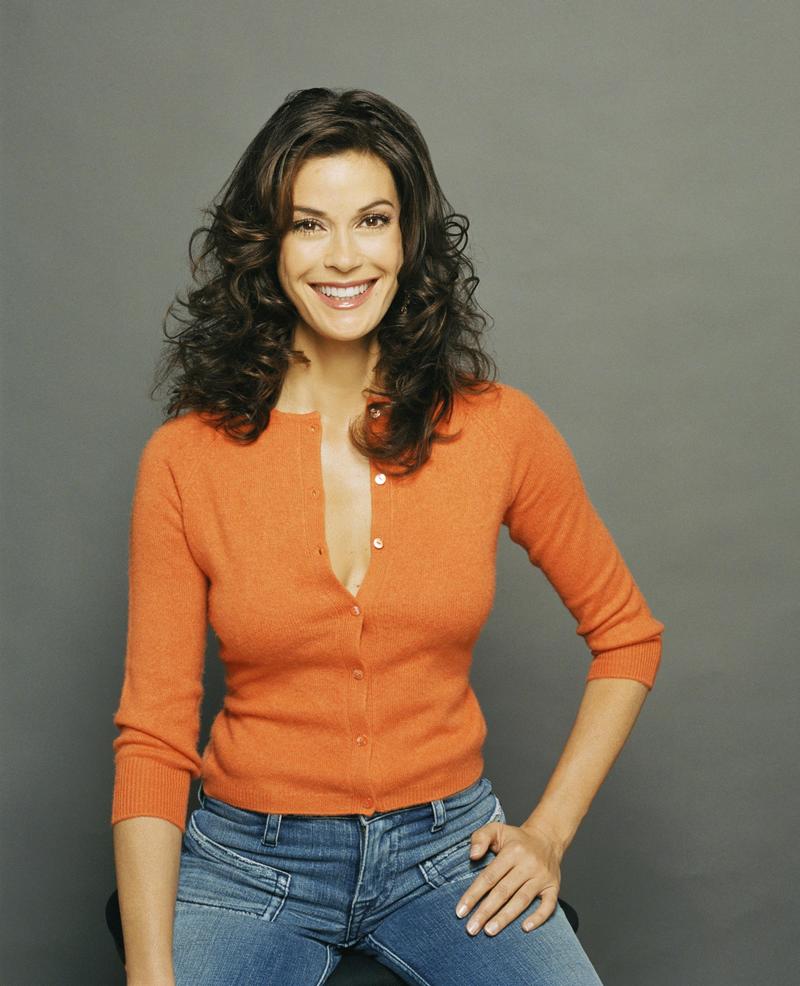The image shows a smiling woman who strongly resembles actress Teri Hatcher, seated on a black stool against a generic gray photographer's backdrop. She has long, wavy brown hair draped over her shoulders, and her expressive brown eyes are looking directly at the camera. The woman is wearing an orange, long-sleeved button-up shirt, which is rolled up to her elbows, partially unbuttoned to reveal a hint of cleavage. Her outfit also includes blue jeans with visible pockets and belt loops. Her left hand is placed on her hip, adding a casual yet confident vibe to the professional glamour shot.